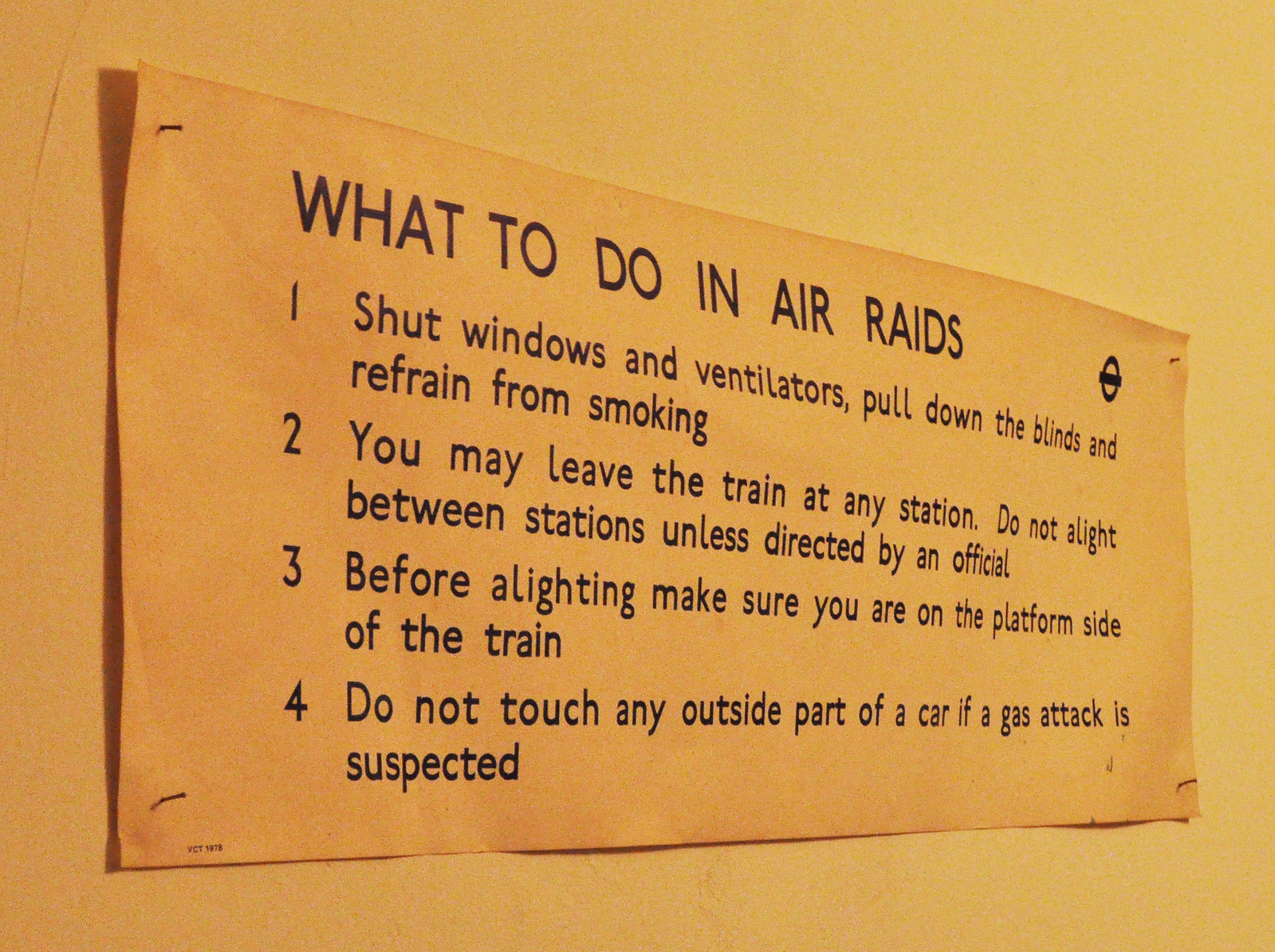This horizontally aligned, color photograph depicts a vintage, slightly curled paper sign tacked to an old, brown background. The sign, positioned centrally, is a landscape-oriented rectangular piece of paper displaying black print that reads, in all caps at the top, "WHAT TO DO IN AIR RAIDS." Beneath this heading, four left-aligned, numbered instructions offer guidelines for air raid safety:

1. Shut windows and ventilators, pull down the blinds, and refrain from smoking.
2. You may leave the train at any station. Do not alight between stations unless directed by an official.
3. Before alighting, make sure you are on the platform side of the train.
4. Do not touch any outside part of a car if a gas attack is suspected.

The background appears to be brown paper attached to another surface, visible through a slit in the upper left-hand corner. There's a small, illegible black logo in a circle in the top right corner of the sign. The overall impression of the image suggests an informational sign preserved in a setting akin to a museum, with the photograph emphasizing the aged and yellowed aspect of both the sign and its surroundings.